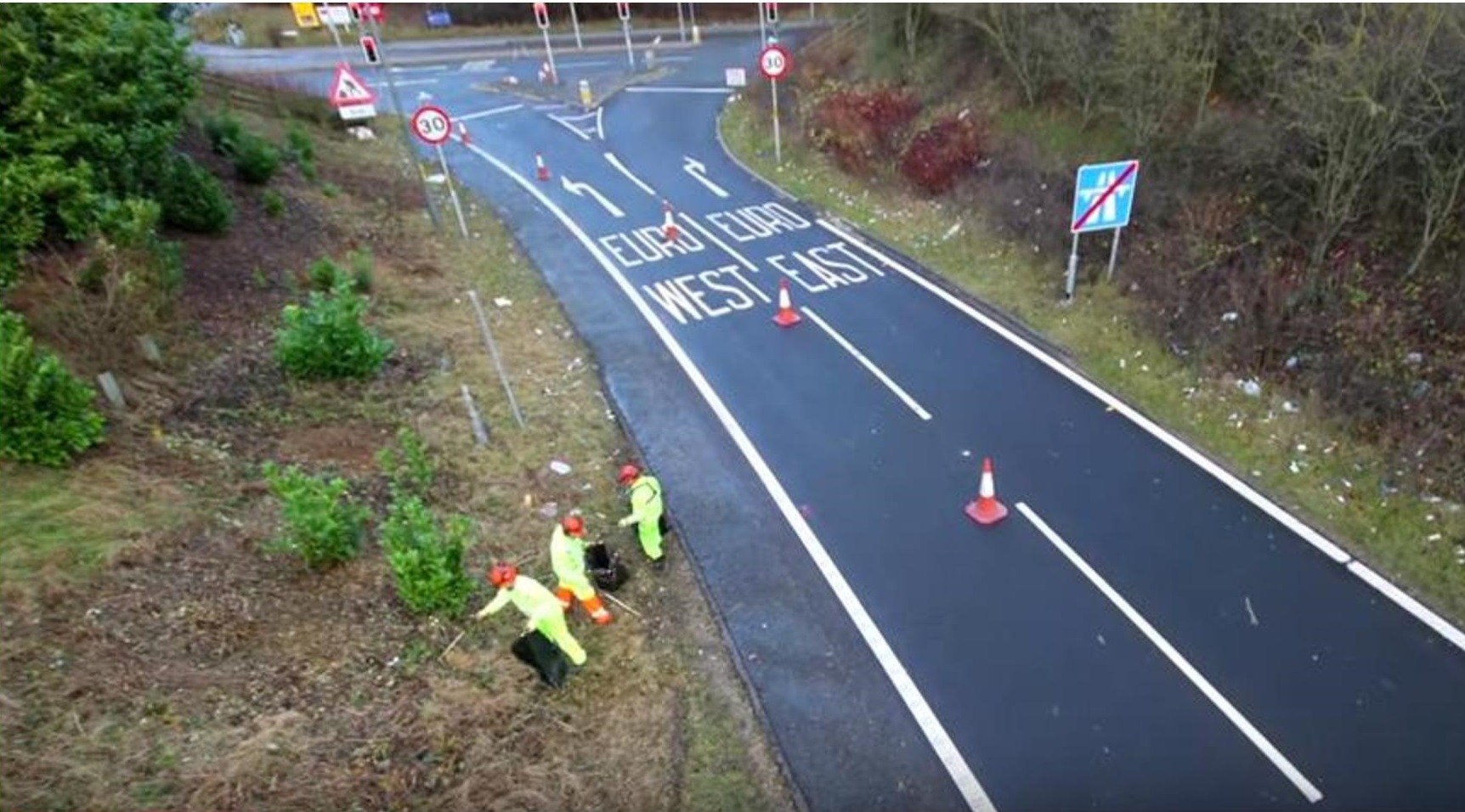The image depicts an intersection of a two-lane road made of black pavement, characterized by solid white lines along the sides and a dotted line dividing the lanes. Red cones are placed down the center of the road. The lanes are annotated with directional labels and arrows: "Euro West" on the left and "Euro East" on the right. There are speed limit signs on each side indicating the number 30. The intersection requires vehicles to turn either right or left, as the road does not continue straight. Grass and trees line both sides of the road. In the center of the image are three workers dressed in high-visibility yellow gear and wearing red hard hats. They appear to be picking up trash, carrying black plastic bags and possibly trash cans. The workers are positioned slightly towards the left and bottom of the center. Streetlights are also visible where the road diverges.